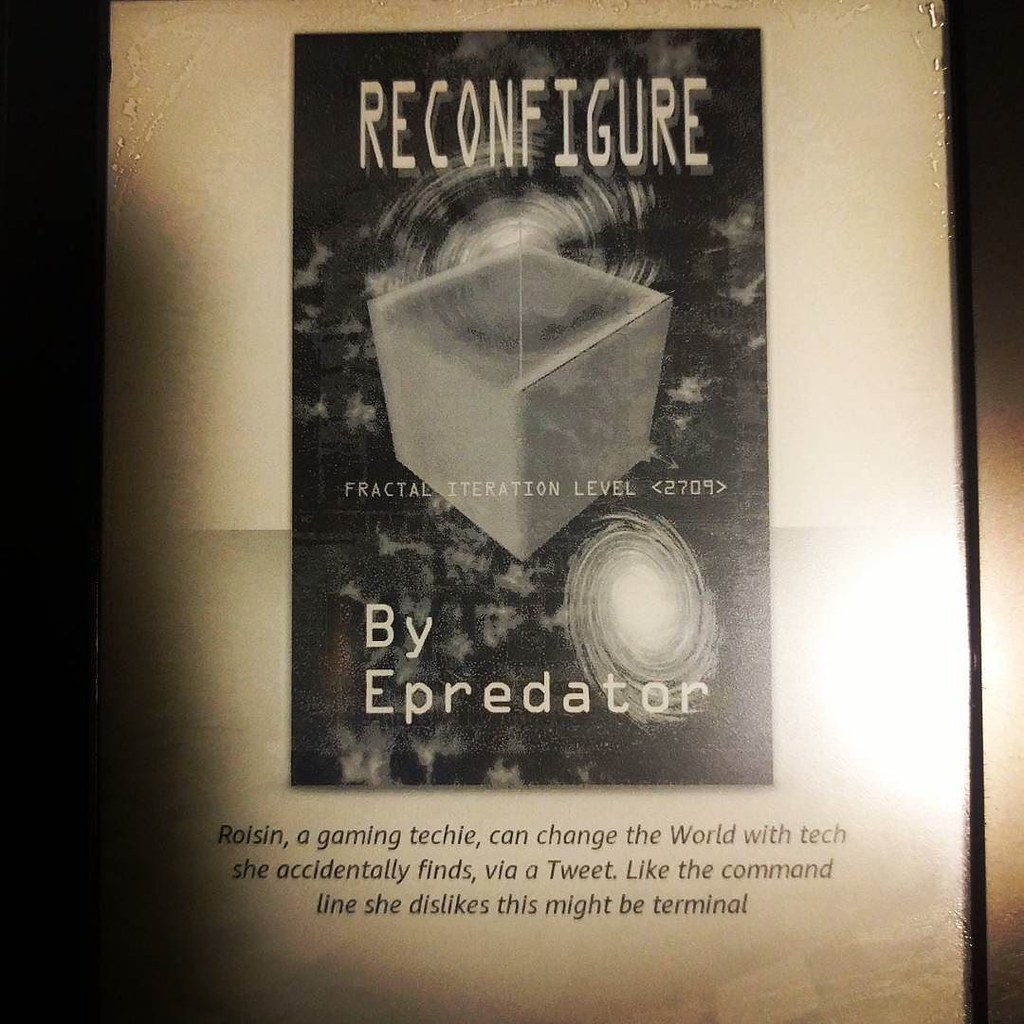The black and white photograph appears to capture the cover of a book titled "Reconfigure" by Efridor. The cover, which sits against a dark cosmic backdrop featuring galaxy-like swirls at the top and bottom right, showcases an intriguing grey cube and a circular, tornado-like design. In bold, white letters, it states "Reconfigure - Fractal Iteration Level 2709" by Epreder. Additional text at the bottom reads: "Royzen, a gaming techie, can change the world with tech she accidentally finds via a tweet. Like the command line she dislikes, this might be terminal." The overall layout and design suggest a 90s tech thriller vibe, and the photo itself resembles a page from a scientific or technical reference book. The photo is vertical, further emphasizing the detailed visual elements of the book cover.